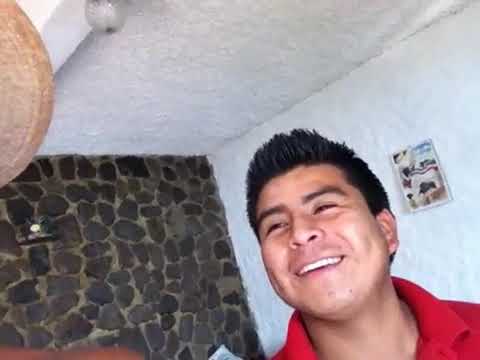The image shows a close-up of a smiling Latin male, identifiable by his short dark black hair and visible teeth. He is wearing a red shirt, with the photo capturing him up to his neck and shirt collar. The background suggests he is in a living space, possibly a living room or a large balcony. One side features a rock-style wall, the rest of the walls and ceiling are white. Behind him, slightly to one side, there's a colorful but indistinct small picture and a lamp in the top left corner. There is also mention of what appears to be another figure with a hat barely visible on the left side. Overall, the scene includes colors like red, white, black, brown, and blue.